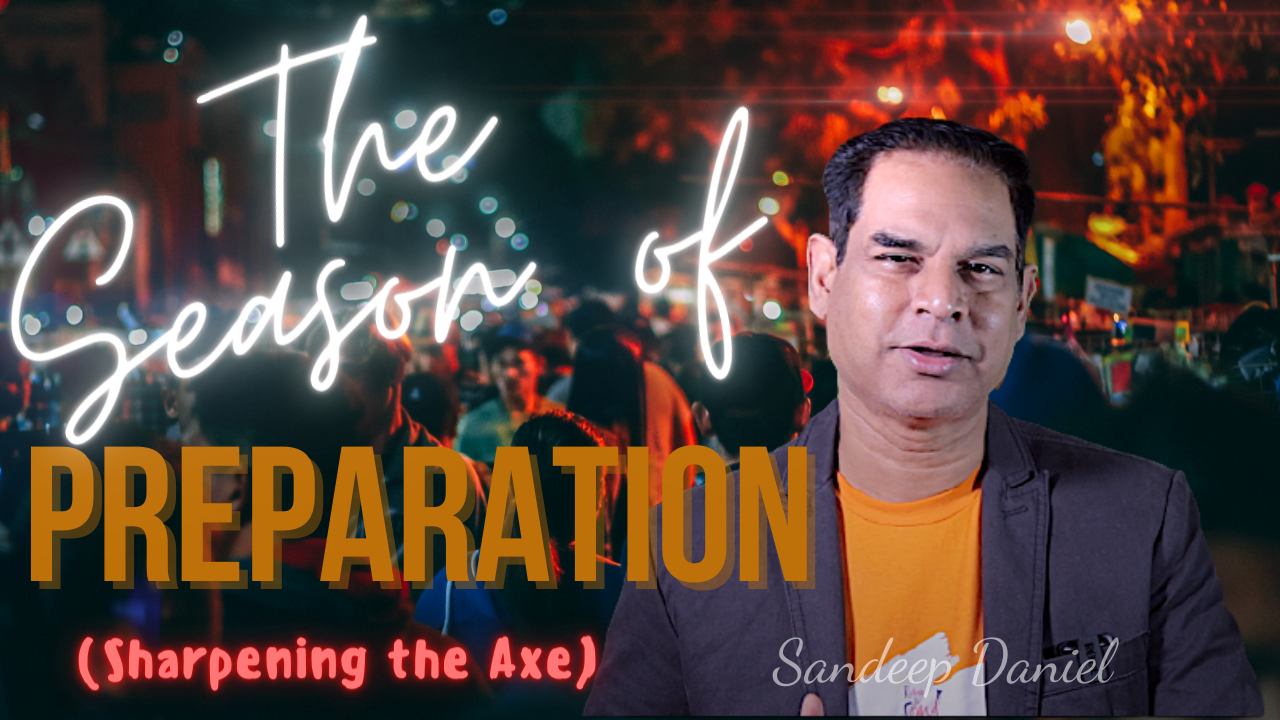The image, likely an advertisement, is a wide, rectangular photo featuring Sandeep Daniel prominently on the right side. Sandeep, presumably in his 40s, has short black hair and dark eyes. He is wearing a dark gray blazer over an orange t-shirt and is looking directly at the camera, his mouth slightly open as if speaking, and his head tilted slightly to the right. At the bottom right, "Sandeep Daniel" is clearly printed. 

The left side of the image contains large, varied font text. "The Season of" is written in bright, cursive white letters, followed by "Preparation" in large, bold burnt orange sans serif font. Beneath that, in a smaller reddish-pink handwritten style, is the phrase "(Sharpening the Axe)." 

The background features a nighttime street scene with various colored lights and blurry, indistinct figures suggesting a party or gathering. The upper right of the image shows trees lit with a red glow, adding to the vivid ambiance of the scene.